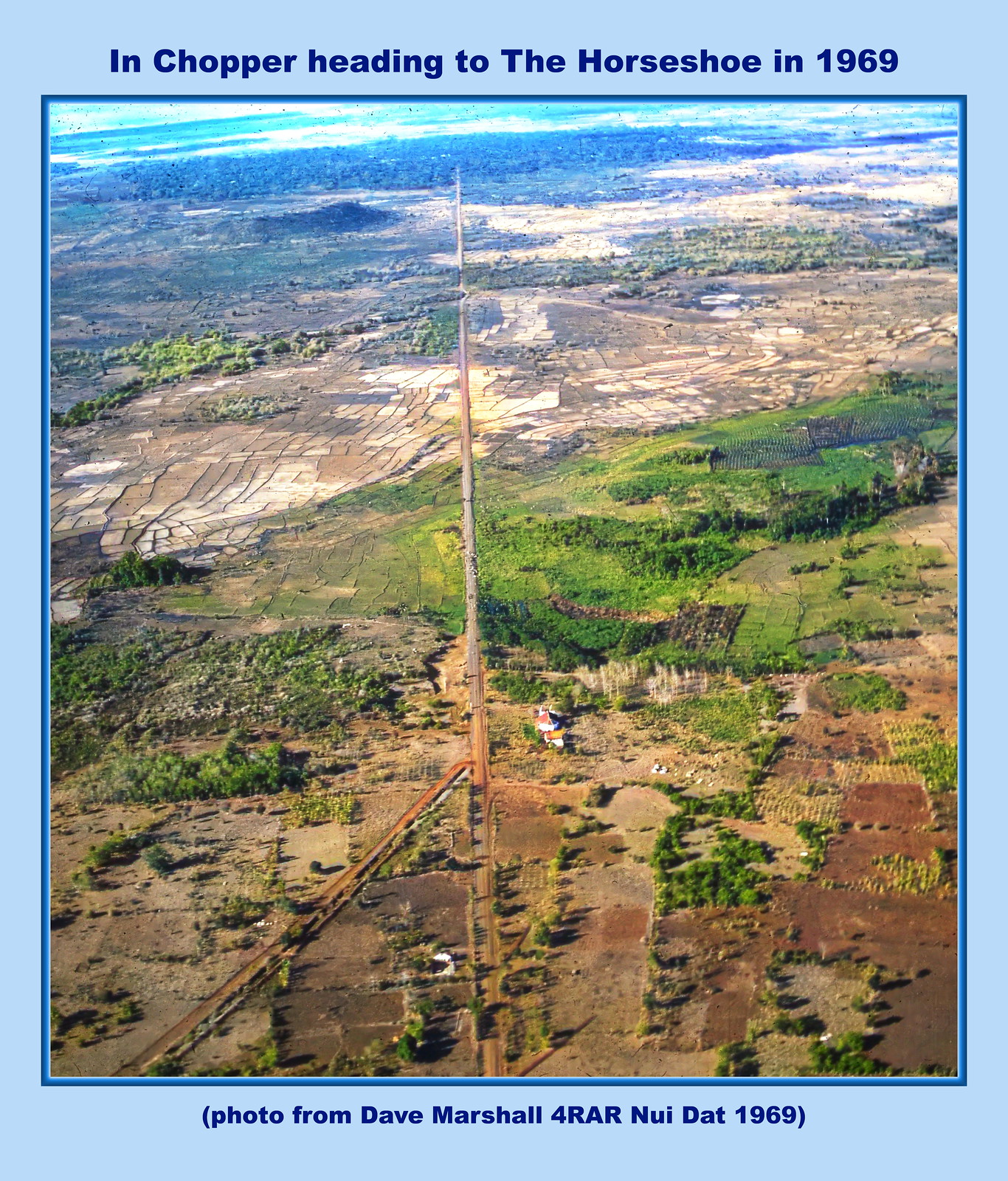This vintage aerial photograph, surrounded by a blue border, displays an extensive overview of Vietnam taken in 1969. The image is captioned at the top with the text "IN CHOPPER HEADING TO THE HORSESHOE IN 1969" and at the bottom with "Photo from Dave Marshall 4RAR, Nui Dat, 1969." The photograph depicts a varied landscape featuring a straight, double-lane dirt road that runs north-south and stretches into a far-off forest, eventually disappearing into the horizon. The terrain consists of a mix of muddy and dry areas interspersed with patches of grass, trees, and agricultural farmlands. Notably, there are also some water bodies and small scattered structures, likely houses, indicating minimal human presence. Despite the greenery and farmlands, the area shows no signs of significant development or population density.